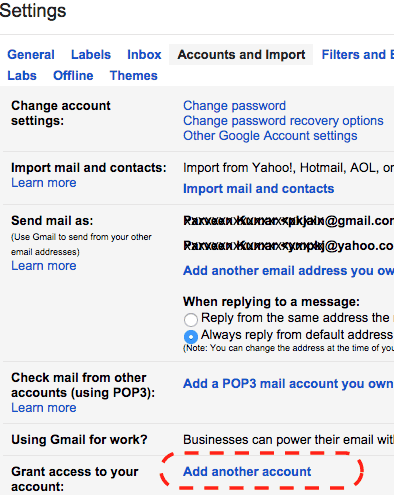This is a detailed screenshot of the Gmail settings interface, specifically taken from a tutorial. The Gmail settings screen is predominantly white, featuring text in both blue and black colors. Positioned in the top left corner is the "Settings" label, followed by various menu options including General, Labels, Inbox, Accounts and Import, Filters, (with the next word cut off), Labs, Offline, and Themes.

The selected menu option is "Accounts and Import," under which several categories and options are displayed. Key elements include:

1. **Change Account Settings**:
   - Change password
   - Change password recovery options
   - Other Google account settings

2. **Import Mail and Contacts**:
   - Import from Yahoo, Hotmail, AOL, or (remainder cut off)
   - A blue button labeled "Import mail and contacts"

3. **Send Mail As**:
   - Use Gmail to send from your other email addresses
   - Two email addresses (one Gmail and one Yahoo), with their details scrambled and X'd out
   - Option to add another email address (partially cut off)
   - Reply from the same address (option cut off)
   - Always reply from the default address (selected)
   - Note about the ability to change the address while composing a message (partially cut off)

4. **Check Mail from Other Accounts (using POP3)**:
   - Add a POP3 mail account you own

5. **Using Gmail for Work**:
   - Business-related email settings (details cut off)

6. **Grant Access to Your Account**:
   - Add another account
   - The "Add another account" hyperlink is circled prominently with a red dashed line.

This detailed setup guides the user through various account and import settings within Gmail, covering essential functionalities like changing passwords, importing emails, sending emails from different addresses, and managing account access.